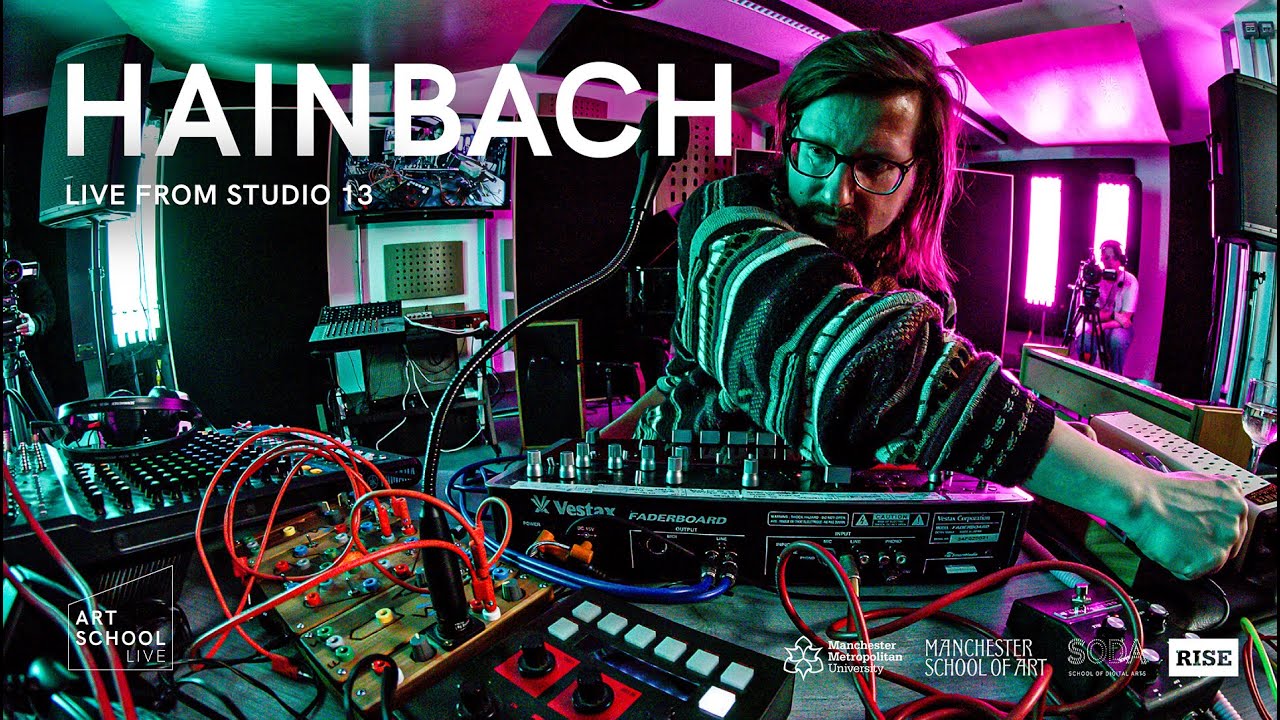This photograph serves as a promotional poster for an event featuring Hainbach, advertised with the text "HAINBACH" in bold, all-caps lettering at the top. Below it, "Live from Studio 13" is displayed in smaller text. The bottom left corner features the label "Art School Live," while the bottom right lists several associated schools: Manchester Metropolitan University, Manchester School of Art, the School of Digital Arts, and something called RISE.

The central figure of the image is a man wearing glasses with black frames, a black-and-white striped knitted sweater, and sporting shoulder-length brown hair, a mustache, and a beard. He is seated at a desk laden with sound equipment, including a complex soundboard with numerous buttons, knobs, and wires. He appears to be in the process of plugging or unplugging wires while intently observing lights on another device nearby. The scene is set in a studio, dimly lit, with a green light illuminating his face. In the background, bathed in pink light, another individual can be seen operating a video camera, capturing the moment.